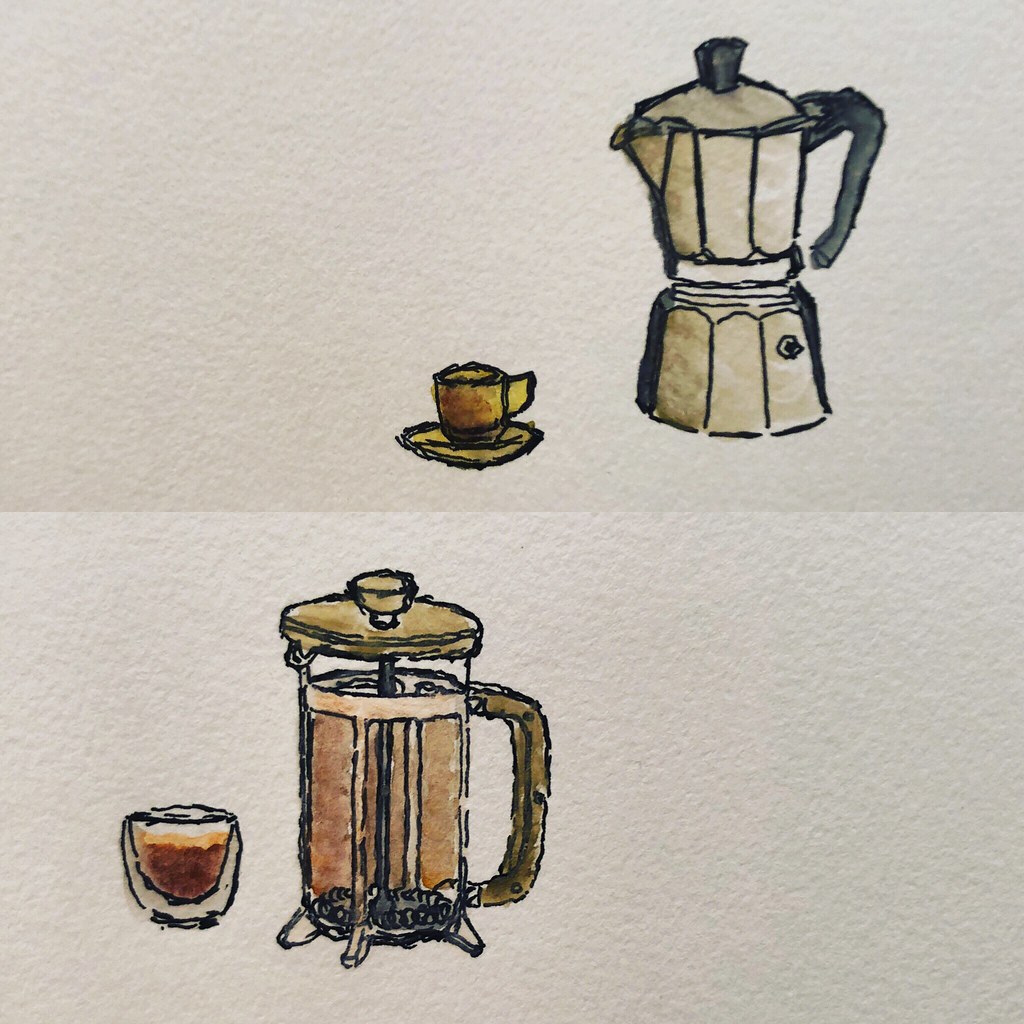The image appears to showcase an artistic assortment of drawings that likely feature teapots and coffee makers, rendered on a piece of white, ruffled cardboard. The paper itself is folded in half, giving it the appearance of a potential greeting card. 

In the top half of the illustration, there is a depiction of a small, yellowish-brown saucer that holds a matching mug. Adjacent to this is a whitish coffee maker or teapot, which is characterized by a black handle and a small switch on its front.

The bottom segment of the card displays a glass mug alongside what resembles the top part of a blender. This blender-like object has a brown handle and a matching brown lid, complete with a knob on top. It appears to be filled with a brown liquid, possibly tea or coffee. The combination of these elements creates a quaint and charming scene, evoking feelings of warmth and homeliness.